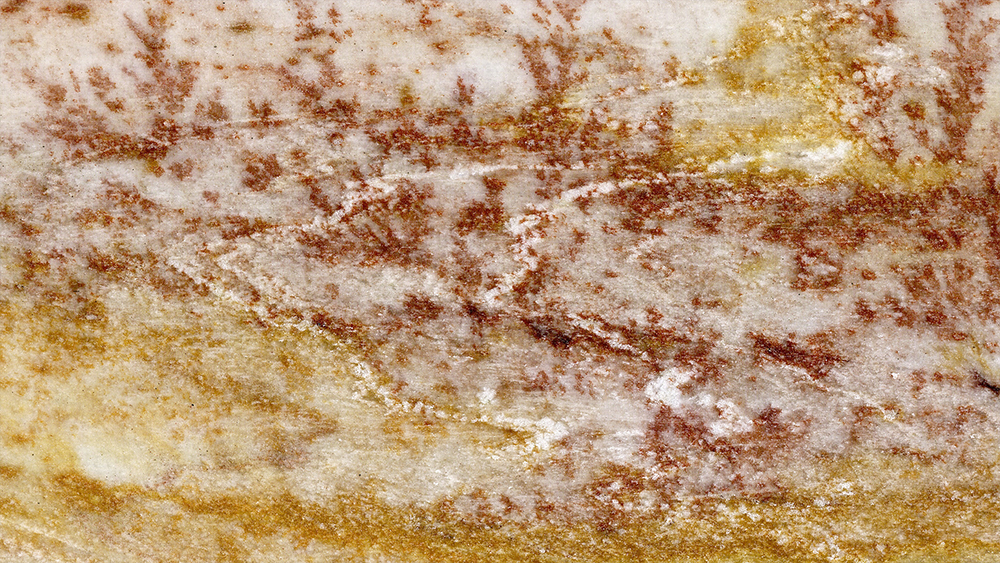This highly detailed color photograph captures an extreme close-up of a piece of limestone, showcasing its complex and varied surface. The rock's texture appears mostly rough with some smoother patches, resembling a dried-out bar of soap. The limestone is a blend of yellow, white, tan, maroon, and brown hues. The bottom section of the rock features a lot more yellow with hints of white, while the middle section contains brown streaks intermingled with faded gray. Notably, the rock exhibits white lines in a wave-like pattern and even triangular formations, with at least two distinct lines and a faint third. These lines form splotches particularly noticeable at the top portion of the image, mixed with a bit of yellow. Near the bottom left corner, a splotchy white area stands out prominently against a cloudy light yellow background. Overall, the limestone's intricate striations and color variations, from dark brown patches to light white veining, are set against a plain white backdrop, emphasizing the rock's natural beauty and unique patterns. The photo is devoid of any people, animals, structures, or motorized vehicles.